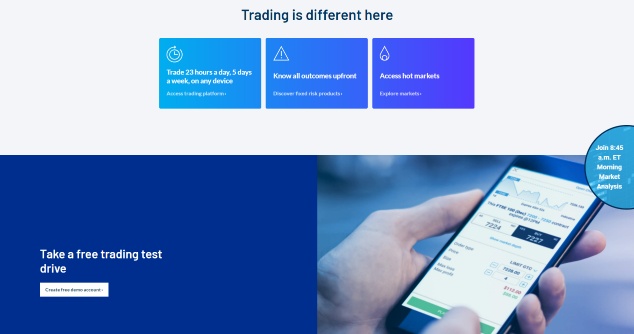In this image, we see a screenshot of a trading website, although the website's name is not visible. The design features a white background at the top and a dark blue background at the bottom. Prominently at the top, a headline reads, "Trading is different here." Underneath, three distinct informational boxes are presented:

1. **Left Box:** "Trade 23 hours a day, 5 days a week, on any device."
2. **Middle Box:** "Know all outcomes upfront."
3. **Right Box:** "Access hot markets."

Towards the bottom of the screenshot, the left side invites users with the message, "Take a free trading test drive." On the right side, there is an image of a man holding a phone, seemingly engaged with a graph, likely for trading purposes. This visual reinforces the platform's utility for active trading and market analysis.

Further down, the text encourages users to "Join H45AMET morning market analysis," promoting an additional feature of the service. The overall intent of the website appears to be to attract users to its trading services, potentially generating revenue through user engagement and advertisements.